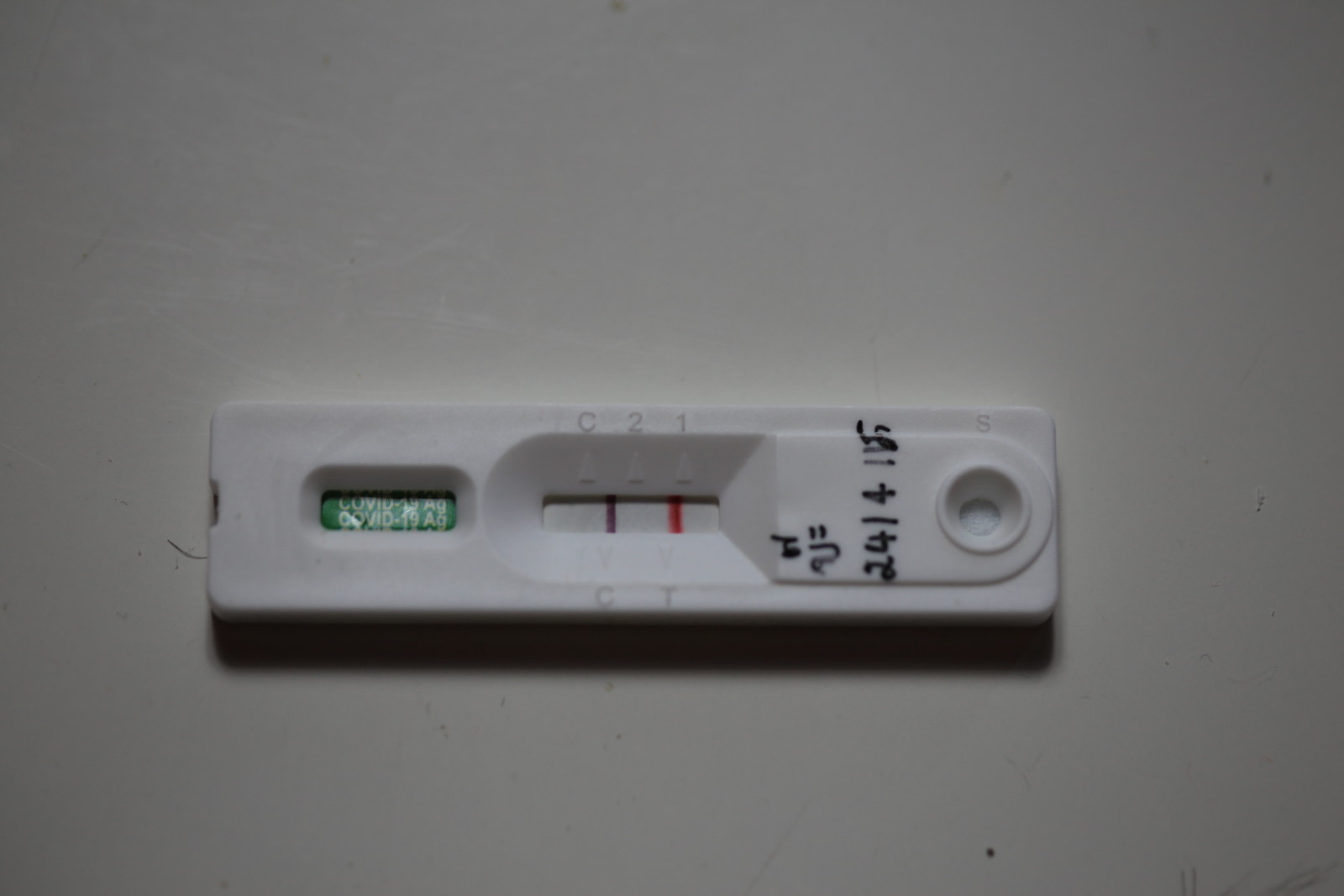This color photograph features a close-up of a COVID-19 test device positioned against a white wall. The test is characterized by its white plastic surface and includes a small window on the left side, labeled "COVID-19 AG" in green lettering. Within the window, a dark purplish line appears, along with a thicker red line to the right. Handwritten numbers, "2414," in black Sharpie, mark the right side of the test. 

The white wall backdrop is slightly marred by subtle scratches and marks, including a small black speck near the bottom right corner, likely dust or dirt. Additionally, a hair can be seen stuck to the left side of the test. The object casts a faint, darker shadow beneath it, adding depth to the otherwise plain white surface.